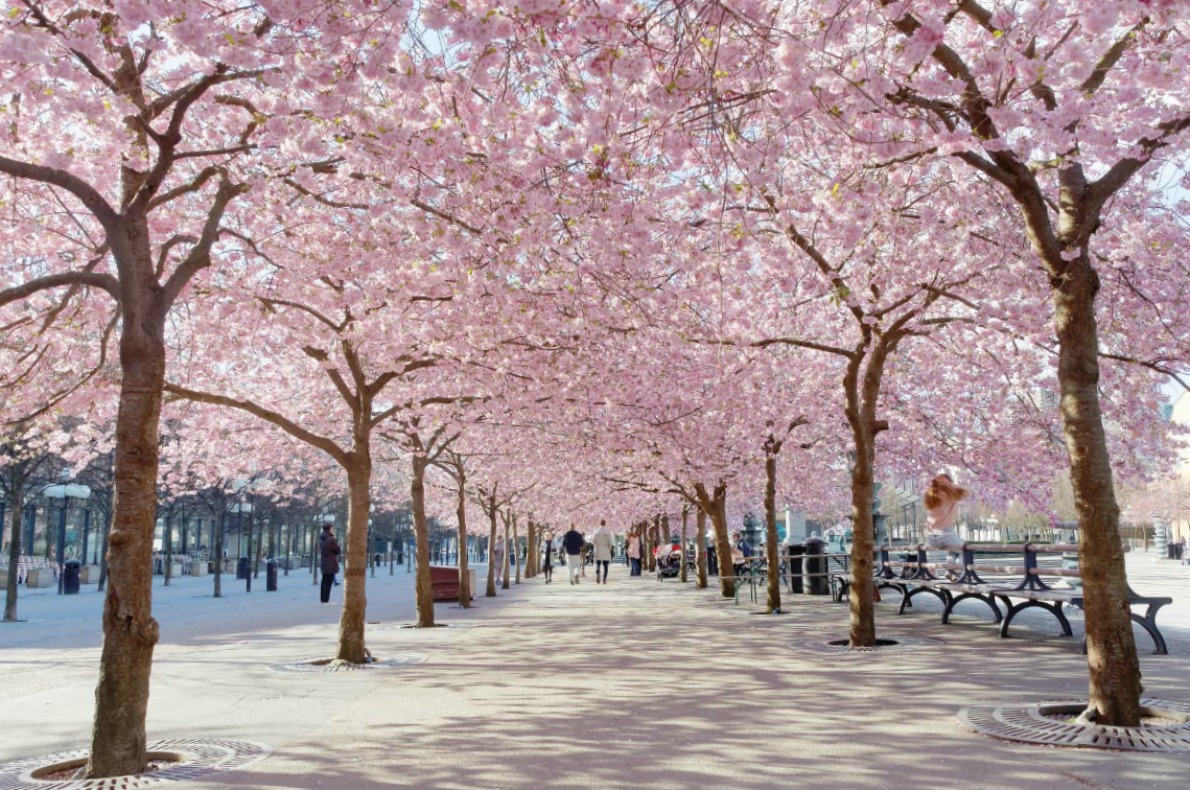This photograph depicts a picturesque urban park scene, featuring an inviting pathway flanked by symmetrical rows of cherry blossom trees. Rising from soil-filled grates embedded in the concrete, the trees arch overhead, forming a stunning canopy of pink blossoms. Sunlight filters down, casting a warm glow on the pathway below, where several picnic tables and lampposts are visible. People stroll through the tunnel-like passage, enjoying the serene beauty of the cherry blossoms. This creates a visually captivating blend of urban infrastructure and natural splendor, with the vibrant pink of the blossoms serving as the focal point.